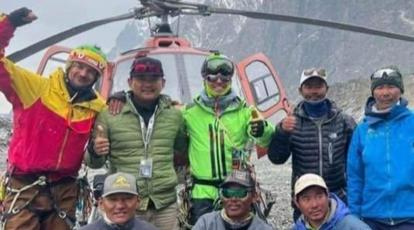This detailed image captures eight men posing in front of an orange helicopter with both doors open, situated on a mountainside. The men are outfitted in a variety of warm jackets, coats, hats, and gloves, indicating they are prepared for cold weather, despite the area having minimal snow. Some men have goggles and sunglasses, and several are giving thumbs up or waving, suggesting a celebratory moment. The backdrop features a steep mountain with patches of snow and rock, along with some plant life on the level area where they stand. Among the group, there are distinct attire differences: two men crouching in front wear gray and blue hoodies, another in the middle sports green goggles, and others are dressed in jackets of yellow and red, green, neon green, a black bubble jacket, and a blue jacket. The orange helicopter with visible propellers and a slightly hazy mountainous background adds to the adventuring spirit captured in this outdoor photograph.